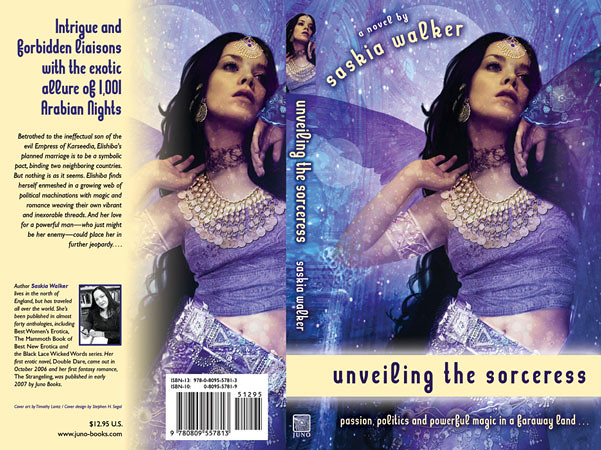This striking book cover, both front and back, is for "Unveiling the Sorceress," a novel by Saskia Walker. The cover art prominently features an enchanting woman who appears to be in mid-dance, dressed in a dazzling, Arabian-inspired outfit consisting of a lacy purple and gold tube top, with a white lacy band around her upper arm. She exudes an air of mystique with her ornate forehead jewelry, long black hair flowing down her back, and gold earrings. Her hands are delicately raised beneath her chin as if she is conjuring magic, enhanced by the seemingly wing-like design behind her, tinged in purple.

The background of the front cover is a mesmerizing swirl of purple and blue, adorned with white star-like flashes, giving a magical, otherworldly feel. Across the top of the cover, it reads "A novel by Saskia Walker," while at the bottom, beneath the title "Unveiling the Sorceress," it states, "Passion, politics, and powerful magic in a faraway land."

The back cover features a continuation of the front cover's artwork, showing the same gypsy-like woman with her intricate jewelry and purple lacy attire. To the left of the image is typical back-cover information, including the title "Intrigue and forbidden liaisons with the exotic allure of 1001 Arabian Nights." Below this, a paragraph provides a brief synopsis of the book's storyline, followed by an author bio accompanied by a black-and-white photograph of Saskia Walker. The back also includes a barcode and the book's price, marked at $12.95 US. This cover beautifully encapsulates the exotic and mystical allure that the novel promises.